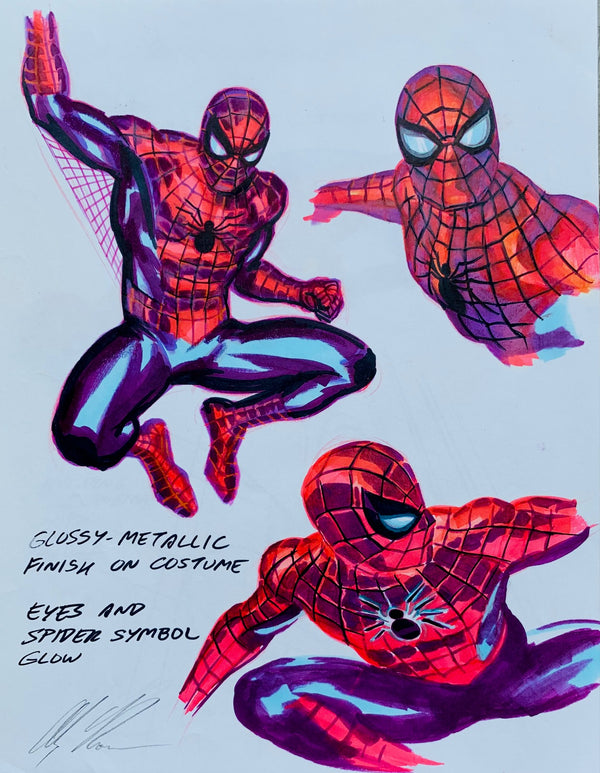This vibrant, hand-drawn cartoon comic book-style painting vividly captures Spider-Man in three dynamic positions against a solid blue background. The largest depiction, in the top left corner, showcases Spider-Man in action: his right arm thrust upwards, his left arm nearly parallel to his bent legs, and he appears to be slinging webs as he looks downward. Directly to the right, a detailed head and shoulder shot reveals Spider-Man's chest emblem and wide-set eyes, as he stares straight ahead. In the bottom right, a profile view shows Spider-Man poised with his arms and legs spread out, in a dynamic, athletic stance, gazing from left to right. Each illustration highlights the character’s signature red and blue suit, emphasized by a polished, glossy metallic finish. A line of text notes how both the eyes and the spider symbol glow. Finally, an illegible cursive signature graces the bottom left corner, authenticating the artwork.